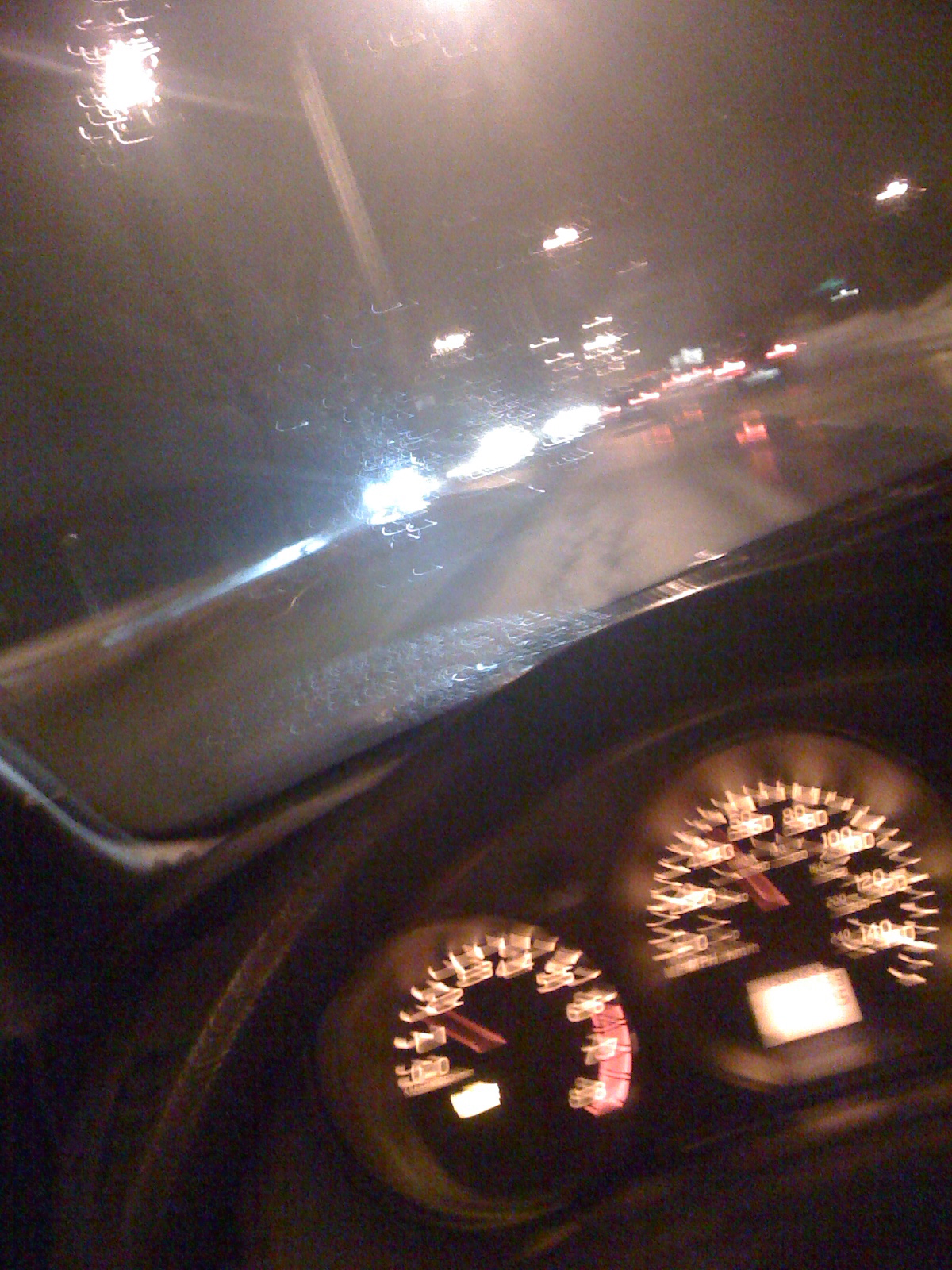A nighttime photograph, captured from the driver's seat of a moving vehicle, features prominently blurred surroundings. The dimly illuminated instrument panel reveals a glowing speedometer and various gauges, indicating the car is in operation. Through the windshield, the cityscape is faintly visible with a smattering of streetlights piercing the darkness. Headlights from oncoming traffic and taillights from vehicles ahead add specks of brightness to the otherwise obscured scene. The pervasive blur challenges the viewer's ability to discern finer details, emphasizing the motion and the nighttime setting of this intriguing snapshot.